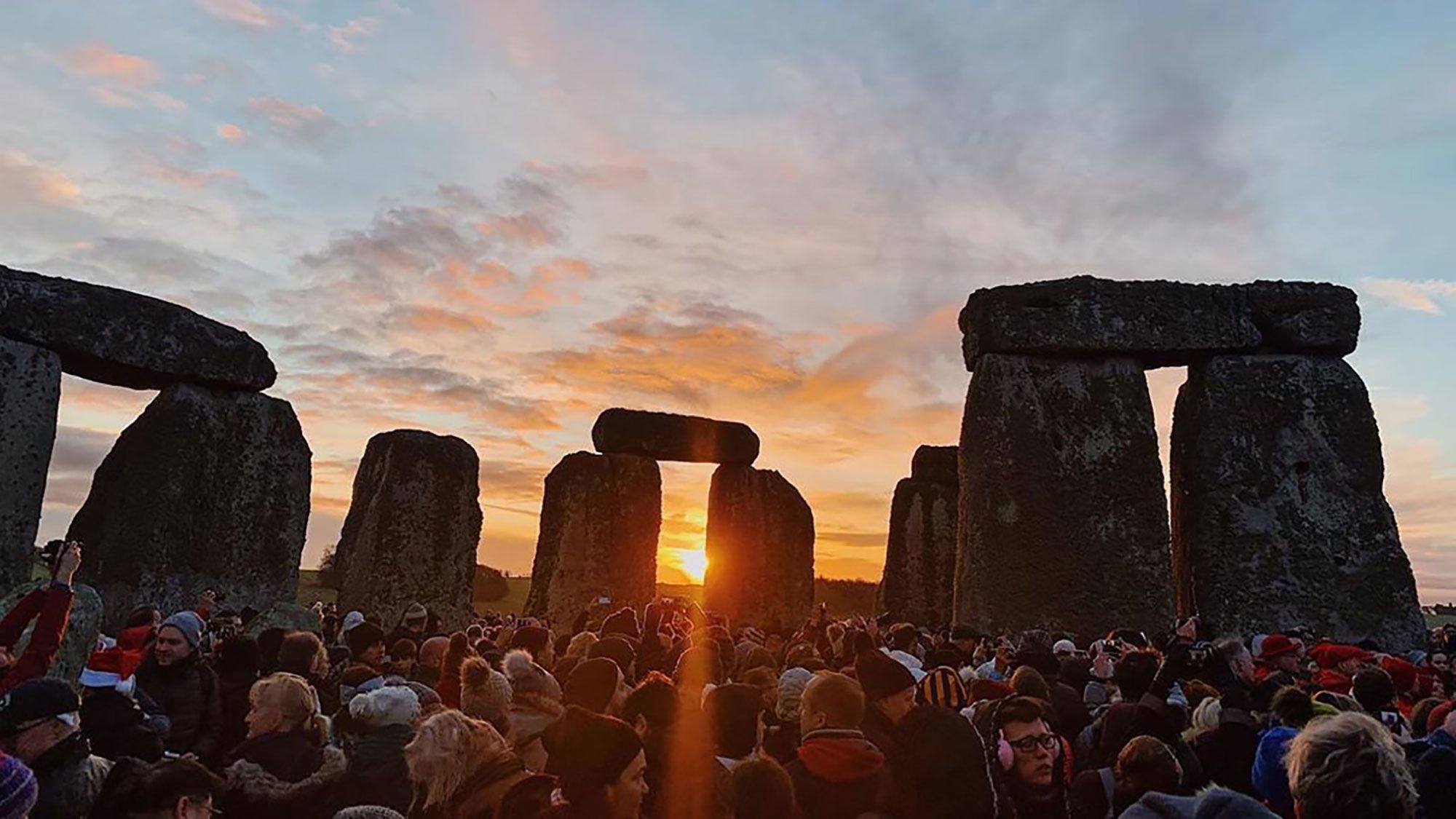This photograph, taken at Stonehenge, captures a striking scene set against the backdrop of either sunrise or sunset. The sky is a blend of light blue with clouds painted in golden pink hues by the sun, positioned just near the horizon. Stonehenge's iconic structures dominate the background, featuring large vertical stones paired with horizontal slabs that span across two vertical pillars, forming several trilithons. There are also a few solitary vertical stones.

In the foreground, a substantial crowd is gathered, suggesting either cold weather or a winter setting based on their attire. The people are bundled in heavy coats, beanies, earmuffs, and some even have blankets, emphasizing the chilly conditions. The diversity of the crowd is notable, with individuals of various ages and races, all enthralled by the ancient monument against the captivatingly warm, orange-tinged sky.